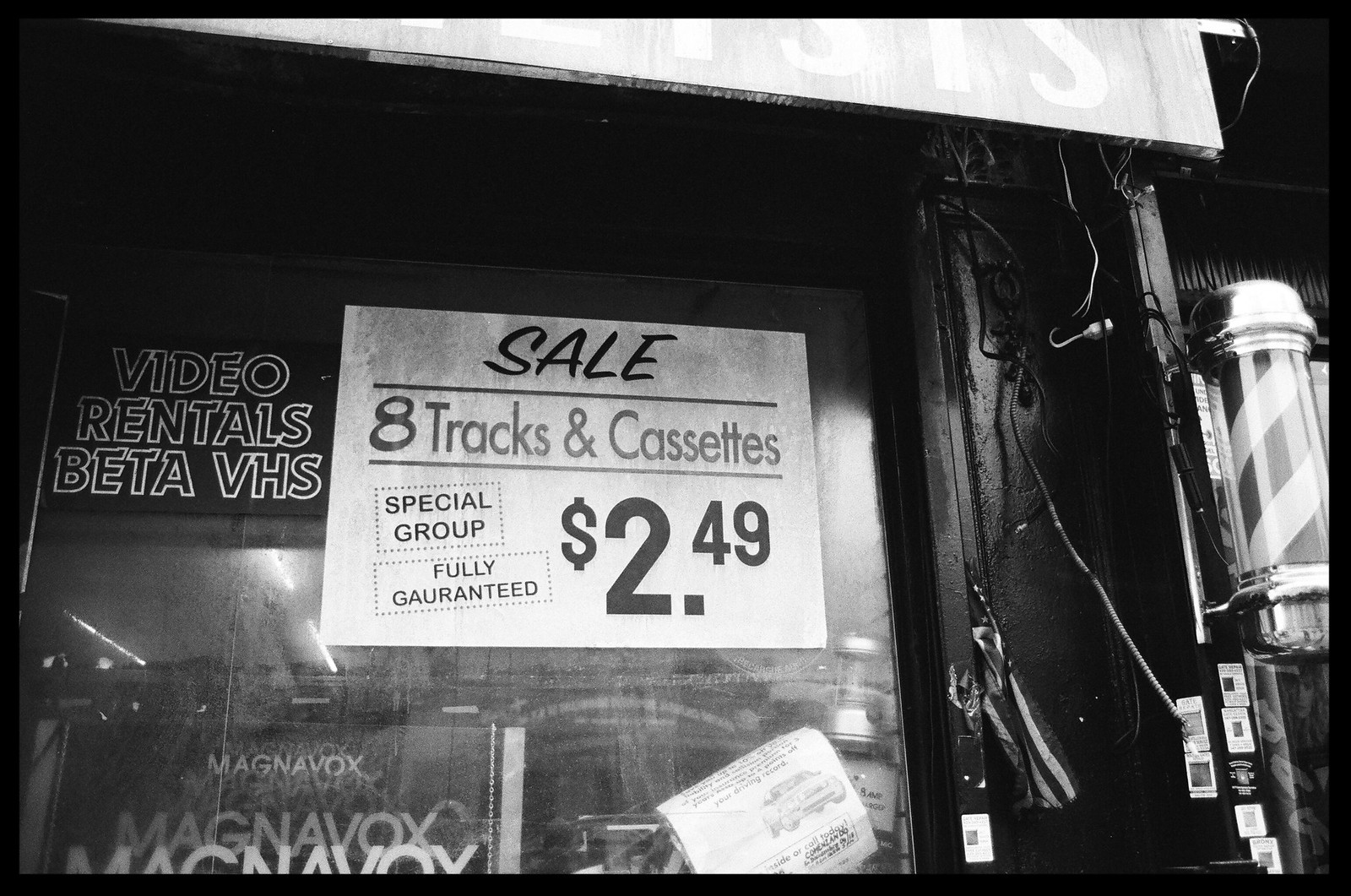This photograph depicts a nostalgic storefront captured entirely in black and white, evoking a moody ambiance where the window area stands out as the brightest part against darker surroundings. The scene prominently features an old camera store's window with vintage signage, including a barbershop pole with red and white stripes on the right side, traditionally indicating that a barber was available. The window itself displays various promotional signs: the upper left reads "Video Rentals, Beta, VHS," and the right side advertises "Sale, 8 Tracks and Cassettes, Special Group, Fully Guaranteed $2.49." The name "Magnavox" is repeatedly reflected in the glass, creating an intriguing visual effect. Despite the monochromatic palette, the intricate details and placement of signs suggest a rich tapestry of mid-20th-century commercial life.